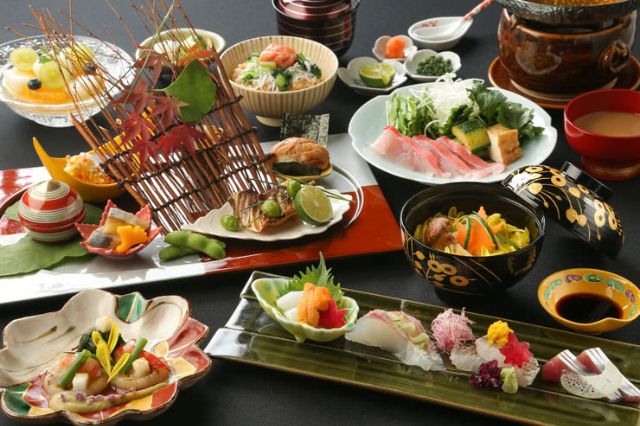On a dark gray slate-colored table, there's a vibrant and detailed array of authentic Japanese dishes. At the center, a long green plate displays an assortment of sushi, accompanied by a small yellow bowl of soy sauce. Nearby, a shell-shaped bowl holds a mix of yellow-green and pink items, possibly a salad. A black bowl with vegetables has its lid slightly ajar, and a white plate features greens and an assortment of sashimi, including white fish and red tuna. A red bowl contains a dark brown soup. A larger rectangular platter showcases grilled fish with decorative elements, bread, limes, and edamame. Additionally, there are dishes of uni (dark orange sea urchin), squid, crab, and various broths, accented by yellow flowers, cilantro, pickled ginger, and scallions. The colorful assortment is arranged in a visually appealing manner with red, white, and yellow plates, making the spread look fresh, bright, and very vibrant.